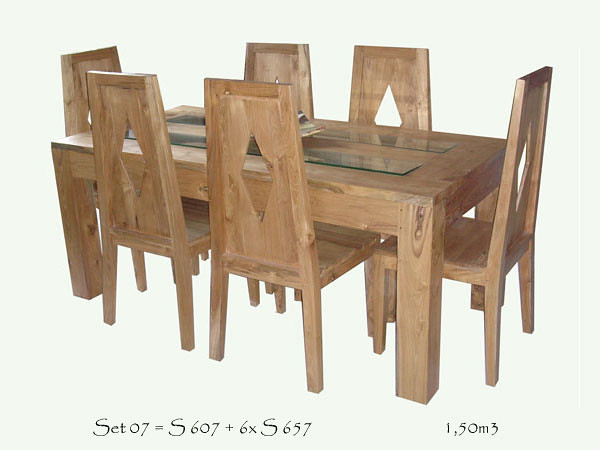This image depicts a rectangular wooden dining table and six matching chairs set against a white background. The table, made from a light to medium brown wood that appears to be either pine or oak, features a large, heavy top inlaid with metal pieces. Additionally, four thin rectangles of glass are set on the table’s surface. The legs of the table are substantial, solid rectangular blocks, providing a sturdy base. Around the table are six chairs, each constructed from the same wood as the table. The chairs have solid backs with distinctive diamond-shaped cutouts for a touch of elegance. There are two chairs on each of the longer sides of the table and one chair at each short end. A notable detail in the image is black writing at the bottom, which reads “set 07 equals S607 plus 6 times S657” along with “1,50M3,” indicating the set includes one S607 table and six S657 chairs. Additionally, there is a silver centerpiece, possibly a covered tray, adding a decorative element to the table.